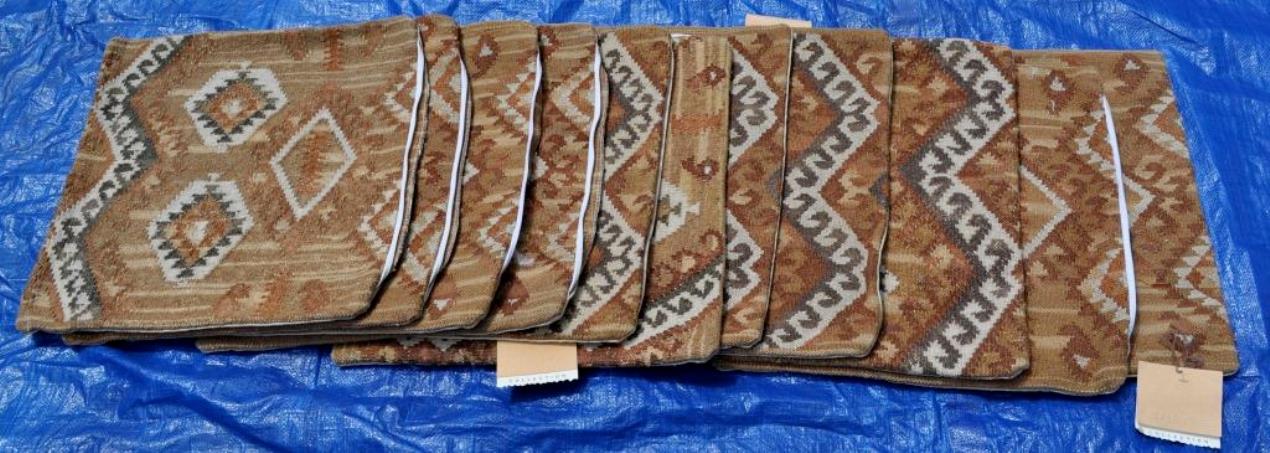This photograph features a series of very thin, square pieces of fabric or possible pillow covers, displayed on a dark blue, slightly wrinkled vinyl tarp that serves as the background. Approximately nine to twelve pieces are laid out, overlapping slightly from right to left, each showcasing a light brown base adorned with various abstract patterns. The patterns exhibit an array of zigzags, diamonds, and dots, using a palette that includes dark brown, black, white, purple-black, and tannish red. Some designs evoke the style of native art or a western horse blanket, while others resemble abstract faces with jagged eyebrows and diamond-shaped eyes. Cream-colored tags and white zippers are visible on some of the pieces, hinting at their function as covers, possibly for pillows. The fabric's artistic motifs and the tactile quality of the blue tarp create a visually intriguing composition.